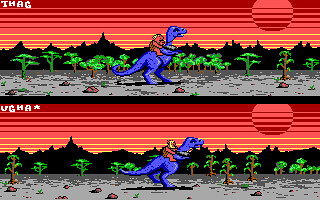The image presents a vividly colored digital scene reminiscent of a classic video game. It is composed of two nearly identical rectangular frames stacked vertically, each showcasing a striking backdrop of bright red with yellow stripes, converging on a large, orange-red sun in the sky to the right. The horizon is marked by a contrasting line of black silhouette trees, adding depth to the colorful panorama.

Stretching across a gray, pixelated ground are several distinct elements: a series of small green plants and shrubs, four prominent red rocks, and a dinosaur traversing the terrain. The dinosaur, varying in description from purple to blue and red, carries a caveman or a character donned in red with a backpack. In each frame, the dinosaur's posture differs slightly, giving an impression of movement. The lush greenery is more pronounced in the upper frame.

Text elements are present in both frames, with "UGHA" featured prominently, albeit split differently across the top left and bottom portions. The carefully crafted scene suggests an adventurous journey set against a captivating, richly hued background, enhanced by its dynamic and whimsical elements.